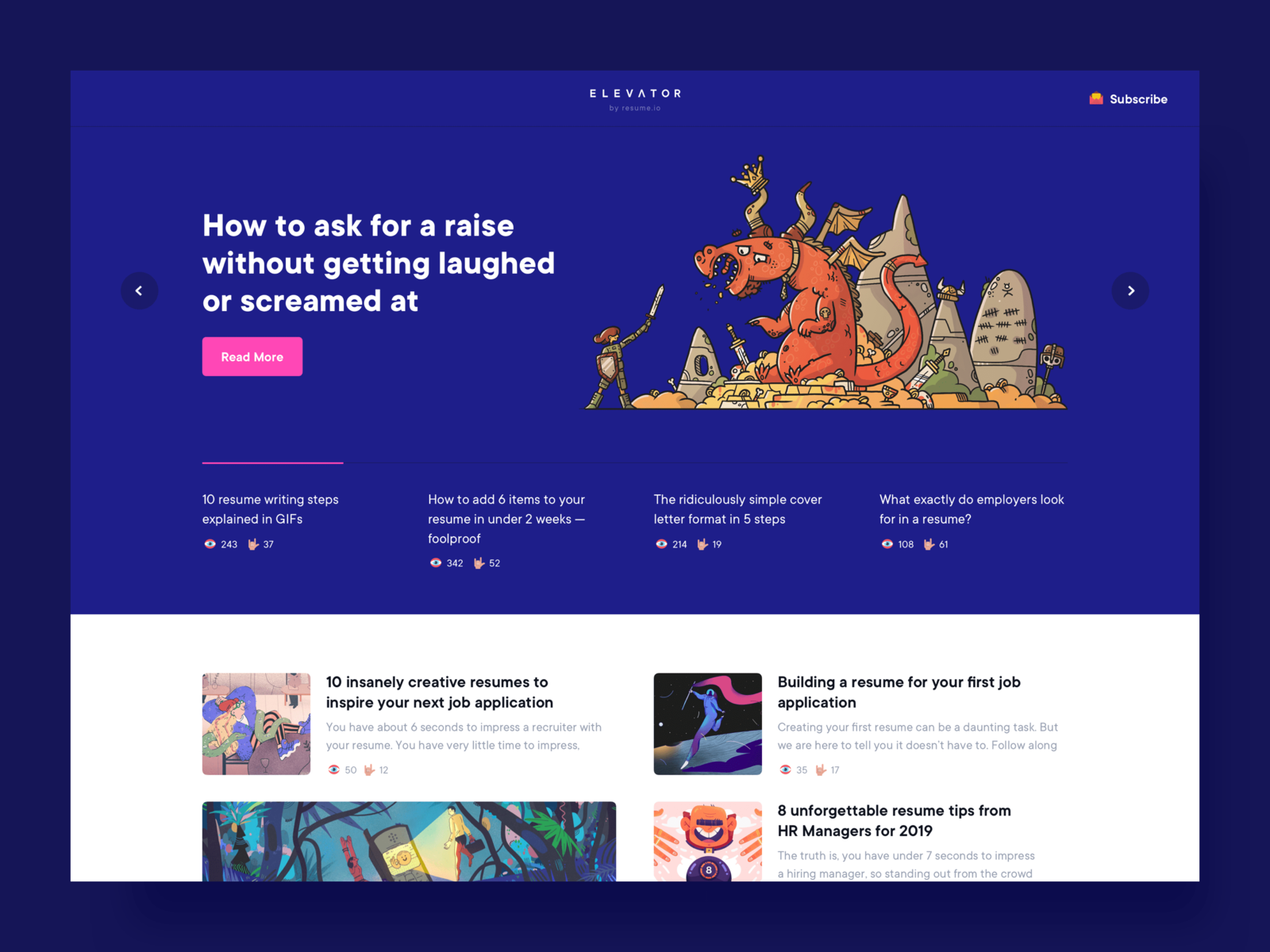The image features a vibrant blue background, prominently centered with a large blue pop-up window. At the top of this window, "Elevator" is written in white font, accompanied by an orange icon and "Subscribe" in white text.

Further down, the pop-up displays the white text "How to Ask for a Raise Without Getting Laughed or Screamed At," followed by a pink and white "Read More" box with a pink underline. Below this, white text lists other articles and resources, including:

- "10 Resume Writing Tips" with an eye icon marked "243" and a hand/leaf icon marked "27."
- "How to Add Six Items to Your Resume in Under Two Weeks - Foolproof," followed by icons and numbers.
- "The Ridiculously Simple Cover Letter Format in Five Steps," with corresponding icons and numbers.
- "What Exactly Do Employers Look for in a Resume," also annotated with icons and numbers.

Above the text, there is an image of a knight with flowing red hair preparing to battle an orange dragon with googly white eyes and tan wings. The scene is surrounded by crumbling gray stone, with a bloody sword stabbed into what appears to be a pile of gold hoarded by the dragon.

Below the knight-and-dragon image, black text reads, "Ten Insanely Creative Resumes to Inspire Your Next Job Application. You Have About Six Seconds to Impress a Recruiter with Your Resume," accompanied by eye and leaf icons.

Continuing down, there's a cartoon-like underwater scene depicting a person approaching a lit-up cell phone, surrounded by brightly colored plants. Following this image is a section titled, "Building a Resume for Your First Job Application," explaining that creating a first resume can be daunting but manageable, with more icons included.

The final partially visible text section, "Eight Unforgettable Resume Tips from HR Managers for 2019," mentions the critical first seven seconds to make an impression, but it abruptly cuts off. Below, there are illustrations of an orange head, orange plants, and a purple eight ball, with no further notable details.